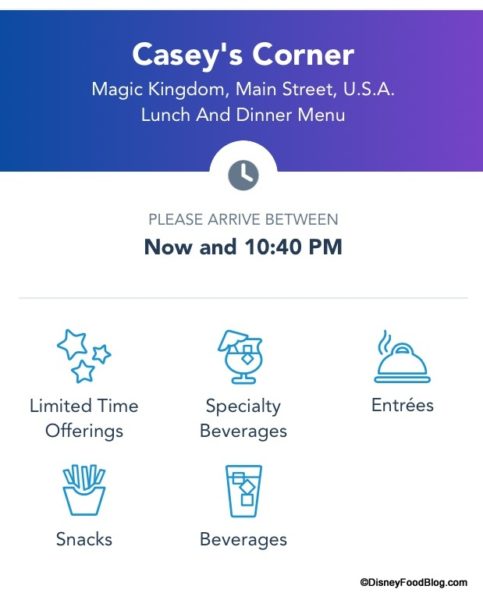The image, captured from a web page, features a detailed header section. At the top, a horizontal blue-purple bar spans the width of the image, with white text that reads "Casey's Corner Magic Kingdom Main Street USA." Directly below that, it states "Lunch and Dinner Menu" in the same white font. Beneath this bar, a gray clock icon is positioned within a gray circle. Following the clock icon, gray text instructs viewers to "please arrive between now and 10:40 p.m." 

A horizontal gray line separates this section from the subsequent details. Starting on the next line, from the left, there are three blue stars labeled "Limited Time Offerings." To the right of the stars, there is a blue outline of a drink, labeled "Specialty Beverages." Adjacent to this, another blue outline depicts a plate and a serving tray, captioned "Entrees." Finally, in the lower-left corner, there is an outline of some chips with the label "Snacks."